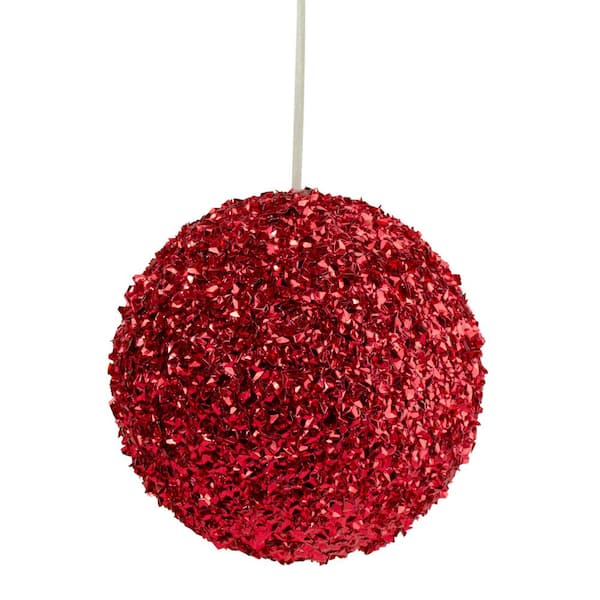The image features an intricate, handcrafted decoration set against an entirely white background. At the center and bottom of the frame, there is a brilliantly bright red spherical ornament. This sphere is constructed from numerous shiny, tinsely particles or strips, giving it a highly textured and crinkly appearance. This tinsel material forms a perfectly round ball that catches light, creating reflections and shadows with some areas appearing darker or black and others lighter red due to the reflective nature of the material. Emerging from the top of this vibrant orb is a thin, white stick or string, adding a final touch to the decoration. The overall impression is of a holiday or arts-and-crafts ornament, with its festive colors and meticulous design, evoking the aesthetic of either a Christmas ornament or a decorative pom-pom.